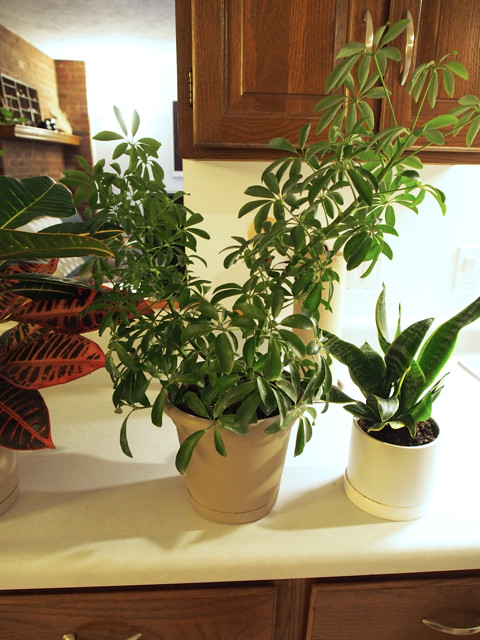This is a detailed colour photograph of an indoor setting, likely a kitchen. Centered on a light beige countertop are two prominent potted plants. The taller plant in the middle is housed in a browny-beige pot, featuring long stems with green leaves that branch out high, particularly to the right. To its right, a smaller snake plant with long, narrow leaves sits in a white pot. On the far left edge of the image, a glimpse of another plant with red and green leaves, likely a coleus, can be seen in an indiscernible pot.

The background reveals elements of a kitchen with upper dark wooden cabinets and lower drawers with visible handles, all in a matching dark wood finish. The wall behind the counter appears light green. A section to the right of the frame hints at another room, showcasing a brown brick wall with a shelf holding various objects, including a small green item and something silvery. Light enters the scene from the right, adding to the bright indoor ambiance.